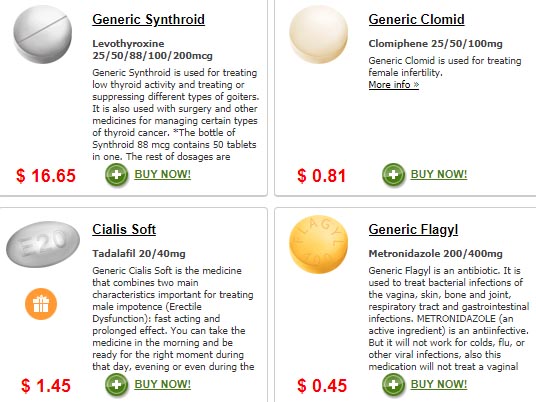This is a cropped screenshot of a pharmaceutical sales web page featuring four products in distinct boxes.

**Top Left Box:**
- **Product:** Generic Synthroid
- **Image:** White pill
- **Details:**
  - Medicine name
  - Available milligrams
  - Description
- **Price:** $16.95, in red text
- **Purchase Option:** Green plus sign and a hyperlinked "Buy Now" in green

**Top Right Box:**
- **Product:** Generic Clomid
- **Image:** White pill
- **Details:**
  - Price: $0.81, in the bottom left
  - "Buy Now" link in the bottom right

**Bottom Left Box:**
- **Product:** Cialis Soft
- **Image:** Oval white pill
- **Details:**
  - Medicine name
  - Available milligrams
  - Description
- **Extra Feature:** Orange box with a white present icon below the pill image
- **Price:** $1.45, in the bottom left
- **Purchase Option:** "Buy Now" link

**Bottom Right Box:**
- **Product:** Generic Flagyl
- **Image:** Yellow pill
- **Details:**
  - Price: $0.45, in the bottom left
  - Description
- **Purchase Option:** "Buy Now" link in the bottom right